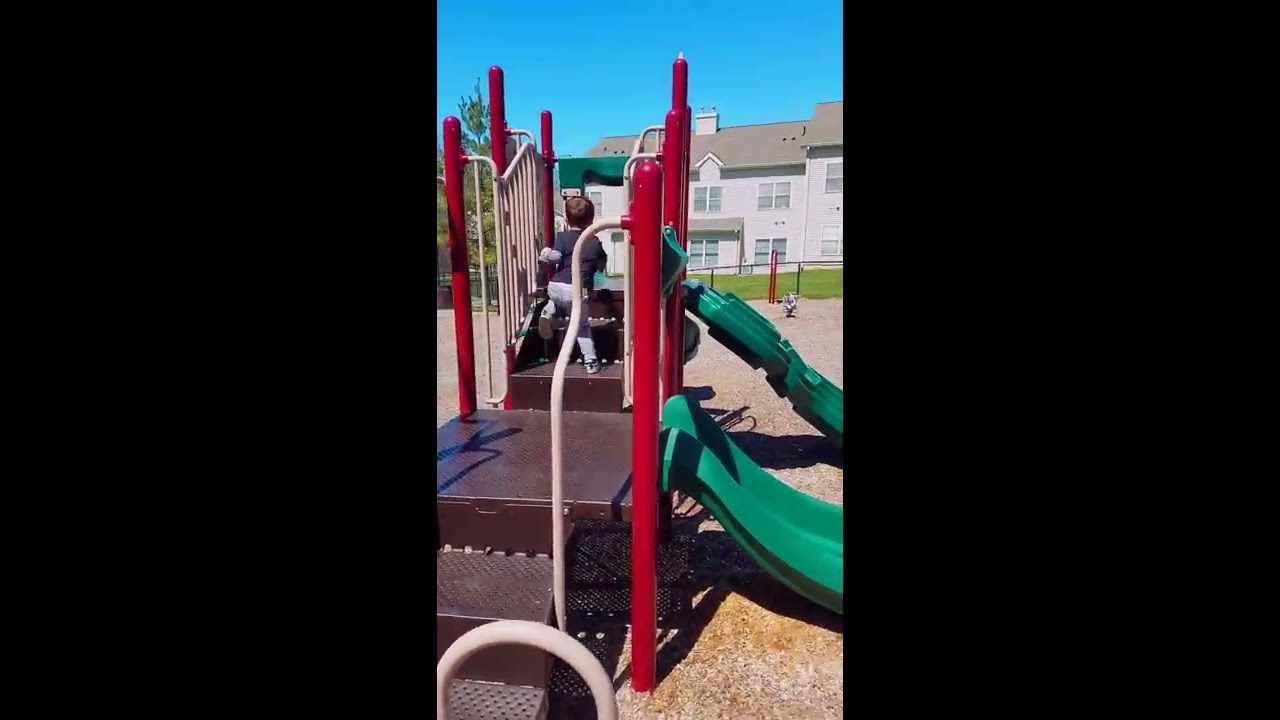The image is divided into three vertical segments, with the left and right segments completely black. The central segment showcases a sunny day with clear blue skies at a playground. Prominently featured is a playscape with a brown stairway leading up to the structure, supported by red columns and enclosed with a white rail. Two green slides extend from the playscape to the ground, which appears to be covered in brownish mulch or pebbles. A young child with brown hair, wearing a dark shirt and gray pants, is seen from behind as he climbs the stairs of the playscape. The setting suggests it is a small, child-friendly playground, bordered by a fenced area with green grass and a two-story building in the background. There are no other children visible, implying the child might be playing alone on this warm, pleasant day.